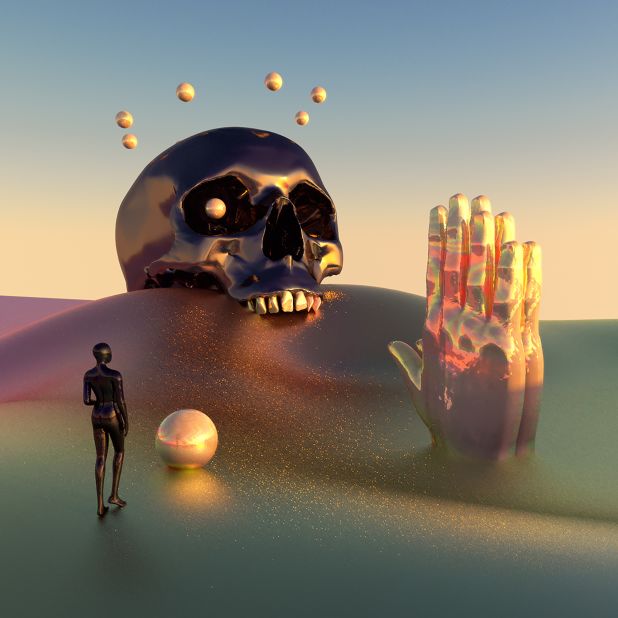This digitally synthesized abstract image portrays a surreal 3D landscape transitioning from a sparkly, rainbow-colored ground at the foreground to a pink and purple hill in the middle. The terrain, appearing both holographic and wave-like with a blend of colors shifting under light, creates a captivating scene. In the bottom left, a featureless, all-black humanoid figure stands nude and hairless, facing away from the viewer. Near its feet is a pearlescent sphere. To the right, two clasped human hands emerge from the ground, adorned in a multicolored, shiny palette including hues of purple, gold, and red. 

Centrally, atop the hill, lies the black upper part of a human skull, featuring golden teeth and a single pearlescent sphere in its left eye socket. Above the skull, six more pearlescent spheres form an outline of a circle. The backdrop of the scene transitions from a warm yellowish-orange near the horizon to a deep blue towards the top, adding to the ethereal atmosphere of the piece.